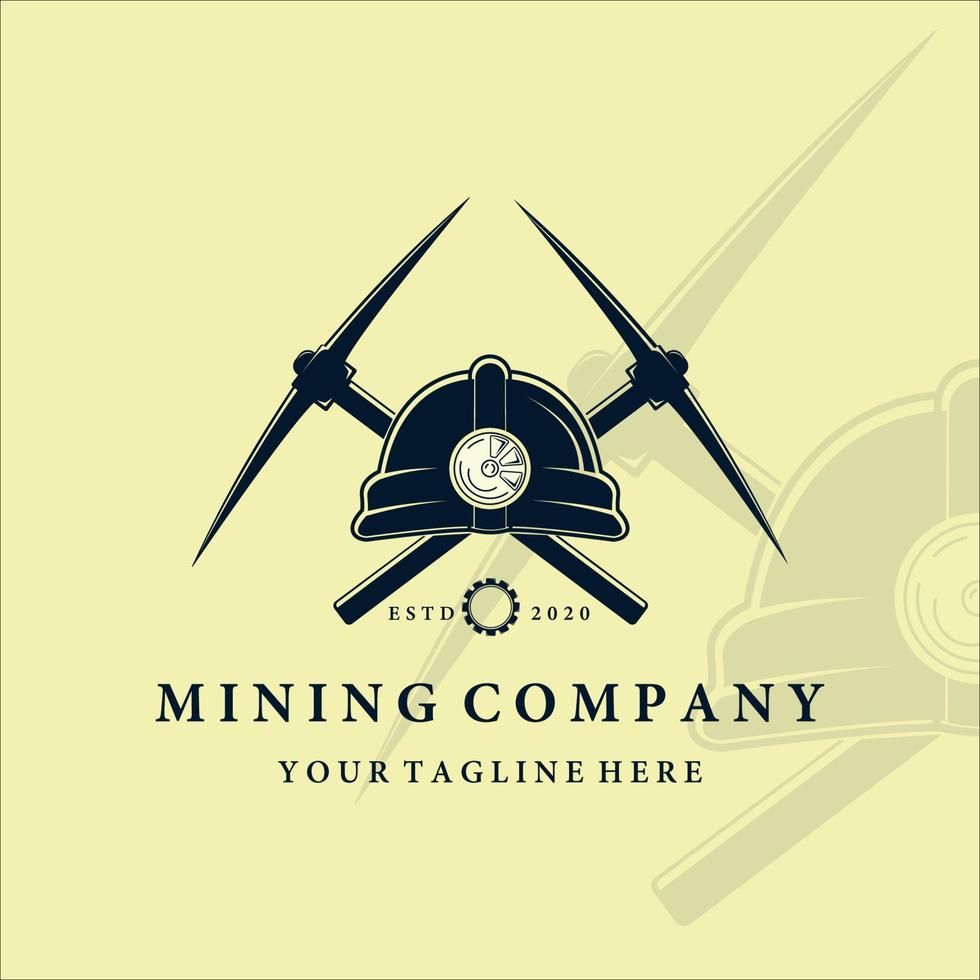The digital image depicts a detailed, created or conceptual logo for a mining company set against a yellowish gray background. Central to the design are two traditional black miner's pickaxes crossed behind a black miner's hard hat, which features a white lamp on the front. Below this emblem, the text "ESTD 2020" is displayed in capital black letters, with the figure "2020" encased in a black circle. Directly beneath this, more black capital letters spell out "MINING COMPANY," followed by "YOUR TAGLINE HERE." Additionally, the image includes a larger, faded, almost ghost-like mirror version of the primary logo in the background to the right, lending depth and shadow to the overall design. The art style is outlined and predominantly black, providing a stark contrast to the muted backdrop.